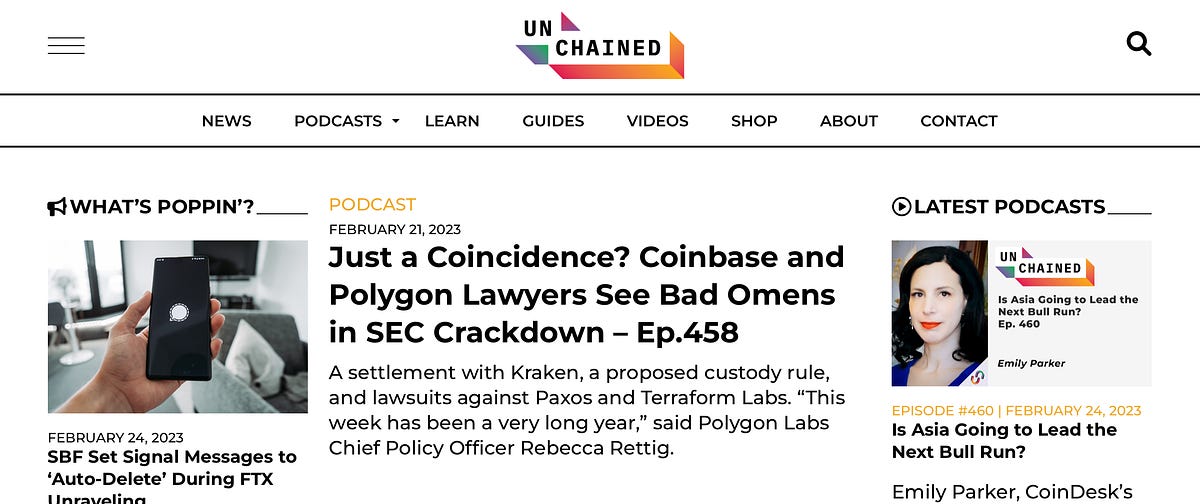This is a detailed description of the home screen for a website called Unchained. The design prominently features isometric cubes in the layout, with the word "Un" positioned in the upper left and "Chained" in the lower right. These cubes are disjointed and connected by angular lines, which are color-graded in shades of blue, red, and orange.

In the top navigation bar, a hamburger menu is located on the left, and a magnifying glass icon for search is on the right. Two thin gray lines frame this menu, which is center-justified and includes options such as News, Podcast, Learn, Guides, Video, Shop, About, and Contact.

The main content area is divided into three columns, with the center column being the widest. 

- The left column features a section titled "What's Popping" accompanied by a megaphone icon, depicting someone holding a phone. Here, a headline reads, "FBF sets signal messages to auto-delete during FTX unraveling."
  
- The center column is dedicated to the podcast section. The highlighted podcast is titled "Just a Coincidence? Coinbase and Polygon Lawyers See Bad Omens in SEC Crackdown" and is labeled as episode 458. Below this, there is additional detailed text likely summarizing the podcast content.

- The right column showcases the latest podcast, featuring a picture of a woman. The headline asks, "Is Asia Going to Lead the Next Bull Run?" and is labeled as episode 460. Next to her photo, the Unchained logo is visible, and the name "Emily Parker from Coindesk" suggests she is the guest speaker on this podcast episode.

This descriptive content effectively conveys the layout, navigation, and key sections of the Unchained website's home screen.